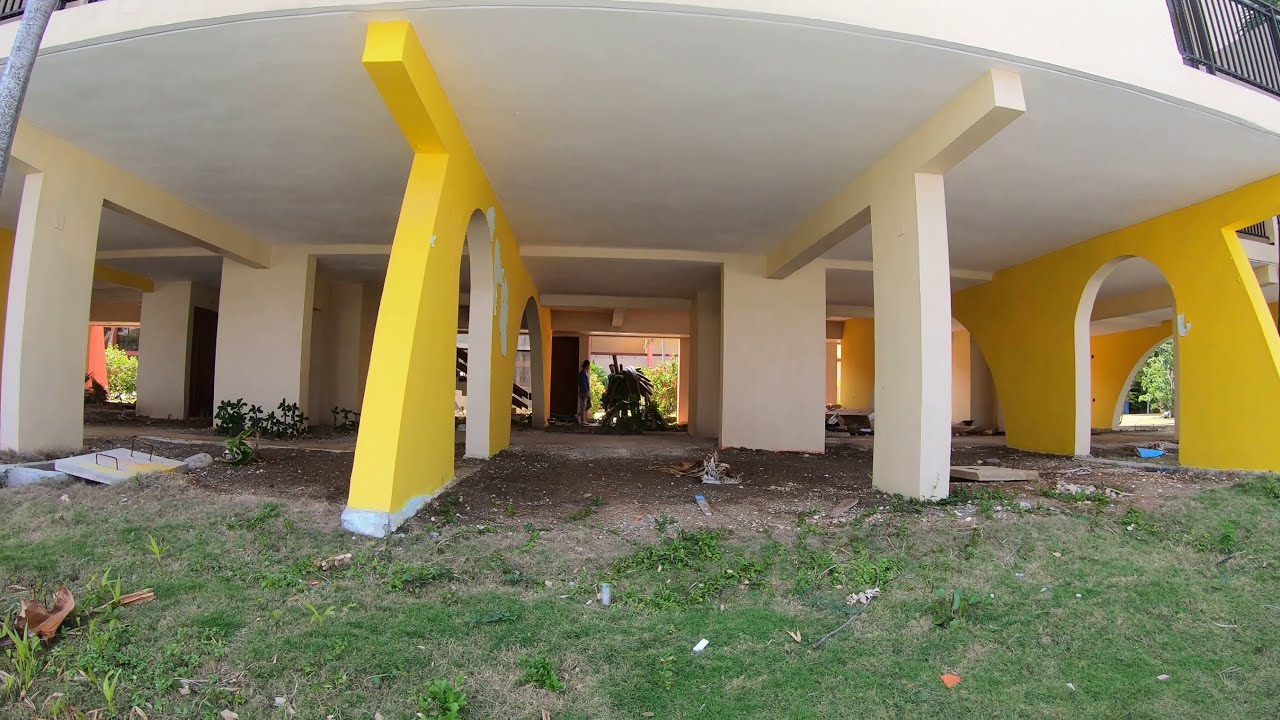In the foreground of the image, a lightly grassed area transitions into a section of bare dirt, leading to the underside of a building that resembles a deck or porch area covering a basement. The understructure is supported by alternating pillars: white square pillars and yellow arches. From left to right, the first pillar is a white square that forms a tunnel-like passage, allowing visibility straight through. Adjacent to it is a yellow arched pillar, followed by another white square pillar forming a T-shaped arch. Towards the right side of the image, two more yellow arches can be seen leading underneath the building, creating a series of tunnels extending back into the structure. The area is sparsely decorated with some pieces of miscellaneous concrete lying around, and in the center, there's a visible doorway and a statue in a lighted area. A black fence runs along the upper floor of the building.